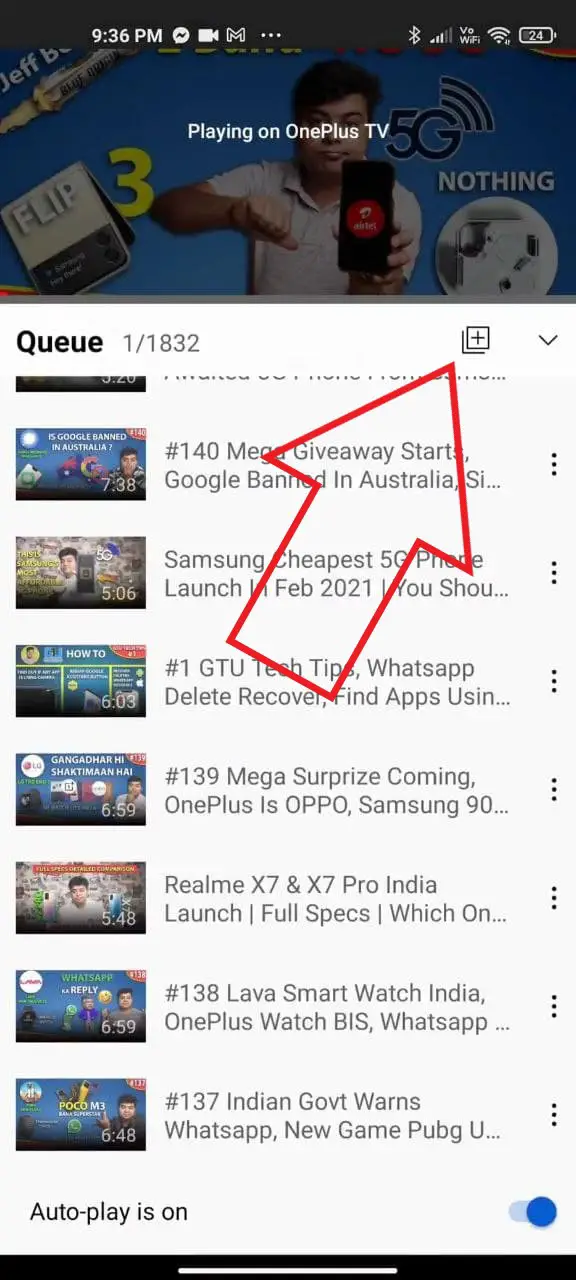The screenshot captures a vibrant section of a website viewed on a phone. The top banner prominently features a man holding a phone, surrounded by various icons including "flip," "nothing," a number "3," a "5G" signal with bars, all indicating different features or concepts. The man is giving a thumbs down gesture. Below this lively banner, the text "Q, 1 out of 1832" is displayed, suggesting a queue or list position.

A large, hollow red arrow points to a plus sign, overlapping some text beneath. The bottom section displays a list of seven items, which appear to be either songs or podcasts, each accompanied by a unique icon and time duration. They include descriptive titles such as:

1. "#140: Mega Giveaway Starts Google Band in Australia."
2. "Samsung's Cheapest 5G Phone Launch in February 2021, You Should..."
3. "#1: GTU Tech Tips – WhatsApp Delete, Recover, Find Apps."

There are four additional entries not fully listed, and the interface indicates that "autoplay is on" at the bottom, concluding with a solid black bar.